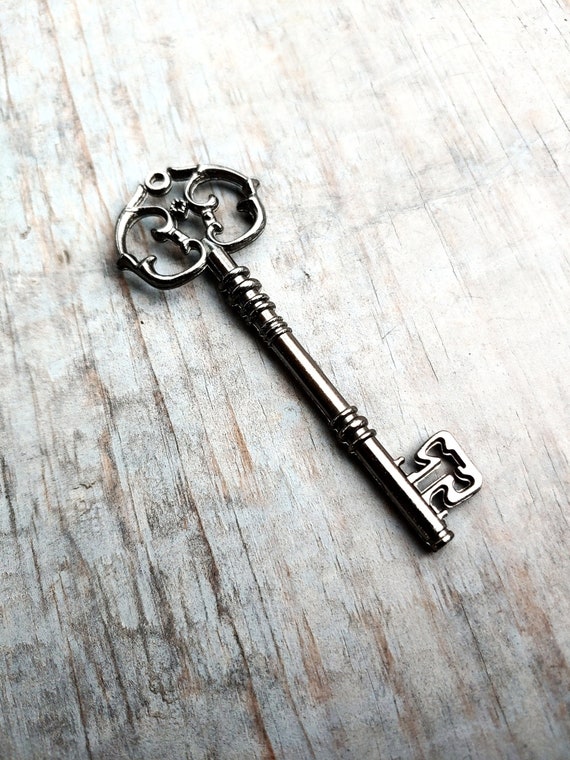The color photograph, oriented in portrait, showcases an intricately designed skeleton key resting on a light wood surface. The wood grain underneath has a mixture of gray and brown hues, emphasizing the earthy and rustic atmosphere. The key itself boasts a light bronze finish with a weathered gunmetal appearance, suggesting it is an aged artifact with antique charm. Unlike modern keys, this key's structure consists of a long, cylindrical shaft adorned with ornamental details, including bands wrapped around its top and bottom. The head of the key features a round design, pointed at the top, and is embellished with symmetrical swirls on either side, resembling a plant pattern. The bottom of the key, reminiscent of an axe head, has two rectangular flaps extending to the right. The key lies at an angle, with its head pointing to the top left and the bottom extending to the bottom right, reflecting light off its detailed grooves and polished surface.